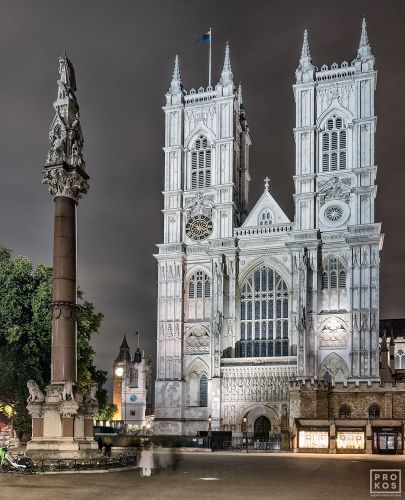The image depicts the majestic facade of Westminster Abbey in London, England, captured at nighttime under a dark gray sky. The grand, grayish stone structure features two towering, Gothic-style spires on either side, intricately adorned with carvings and embellishments. The central part of the cathedral houses a large, arched stained glass window just above the main entrance. Positioned atop the roof's center is a simple cross. Each of the two main towers is flanked by four spires, one at each corner.

In the foreground, there is an expansive plaza with a prominent, rounded base supporting a towering monument. The monument features detailed carvings near its base, with a statue perched on top, almost rivaling the cathedral’s height. To the left of the monument, Big Ben’s iconic clock tower and another white tower can be glimpsed in the background, adding depth to the scene. A flag, possibly the Ukrainian flag with yellow and blue stripes, waves faintly in front of the illuminated cathedral, which stands eerily empty, exuding a serene and timeless aura.